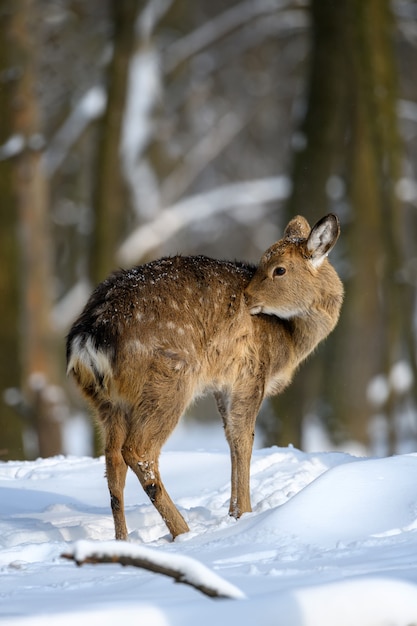The image captures a young deer standing in a snowy forest. The forest background is out of focus with tree trunks subtly visible and snow covering the ground and branches. The deer, with its side profile facing right, turns its head back to nuzzle its shoulder, revealing black eyes and a white-tipped nose. Its fur is predominantly light brown with a dark brown ridge along its back and scattered white spots, hinting at its youth. The tail is mixed black and white, and its ears are black-tipped with white fur inside. A thin layer of snow lightly dusts the deer’s back and head. In the foreground, a snow-covered log is visible, blending into the serene, wintry landscape.